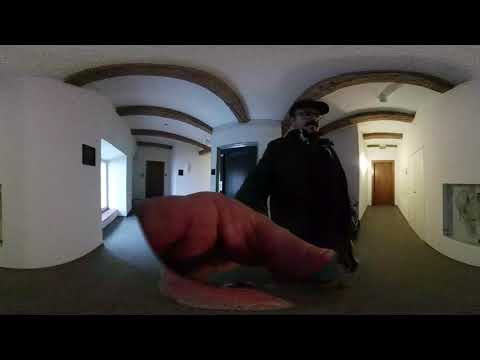The image captures a man walking down a white-paneled hallway with a brown carpet and wooden columns on the vaulted ceiling. He wears a black winter coat, a black baseball cap, glasses, and has a black mustache or goatee. The panoramic nature of the photograph creates a slight distortion, making the hallway appear to curve and partially mirror itself. He carries a red soft material, possibly a blanket. His arm is outstretched towards the camera, creating a distorted view that makes his hand appear unusually large and somewhat disconcerting. Behind him, the hallway extends with white walls, brown doors, a plaque, and at least one painting. There is a window on the left side, allowing daylight to filter in, while the right side appears darker without windows. The unique angles and the distortion of his hand give the scene an almost surreal atmosphere.